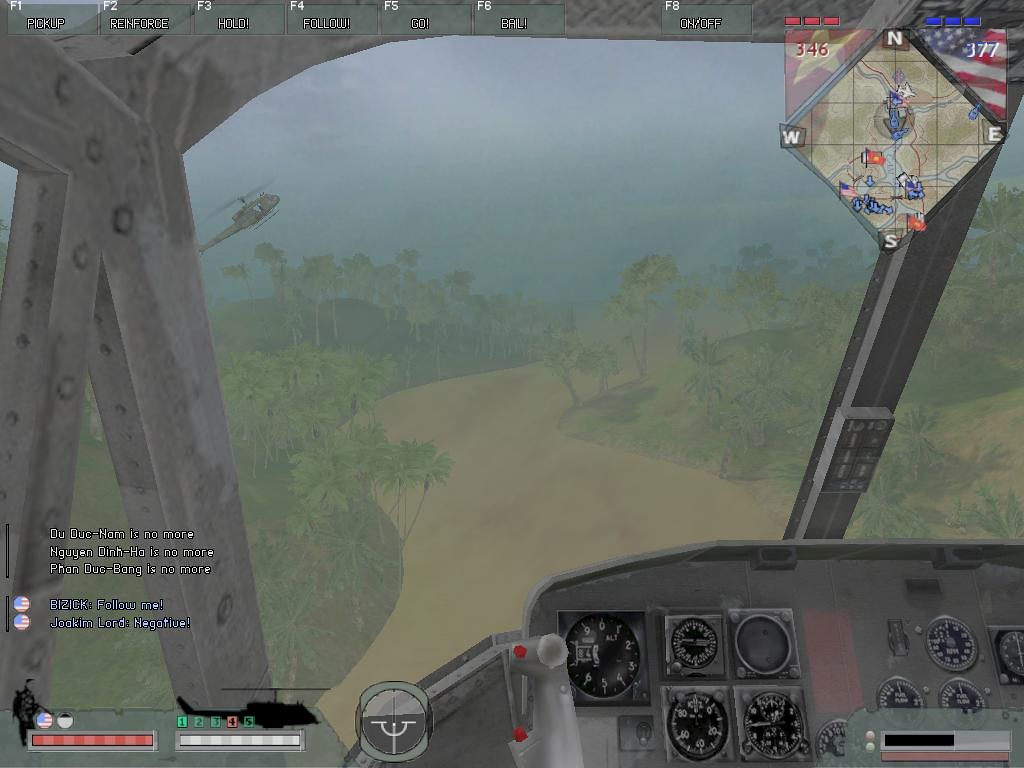The image depicts a highly-detailed helicopter cockpit from a video game. The cockpit is equipped with various controls and gauges, primarily in black and white, offering a realistic and immersive flight simulation experience. In the bottom left corner of the screen, a red health bar and a fully-charged white bar provide vital status information. Above these bars, several lines of text read: "Dooduck Nom is no more, Nagoyan Dink Ho is no more, Fuckin Do Bang is no more, Bizik Follow Me, Joe Kim Lord, Negative." Notably, an American flag is displayed next to the names Joe Kim Lord and Negative. In the top right corner, a small map assists with navigation, also marked by an American flag. The background reveals another helicopter flying over a lush jungle landscape, adding depth and context to the scene.